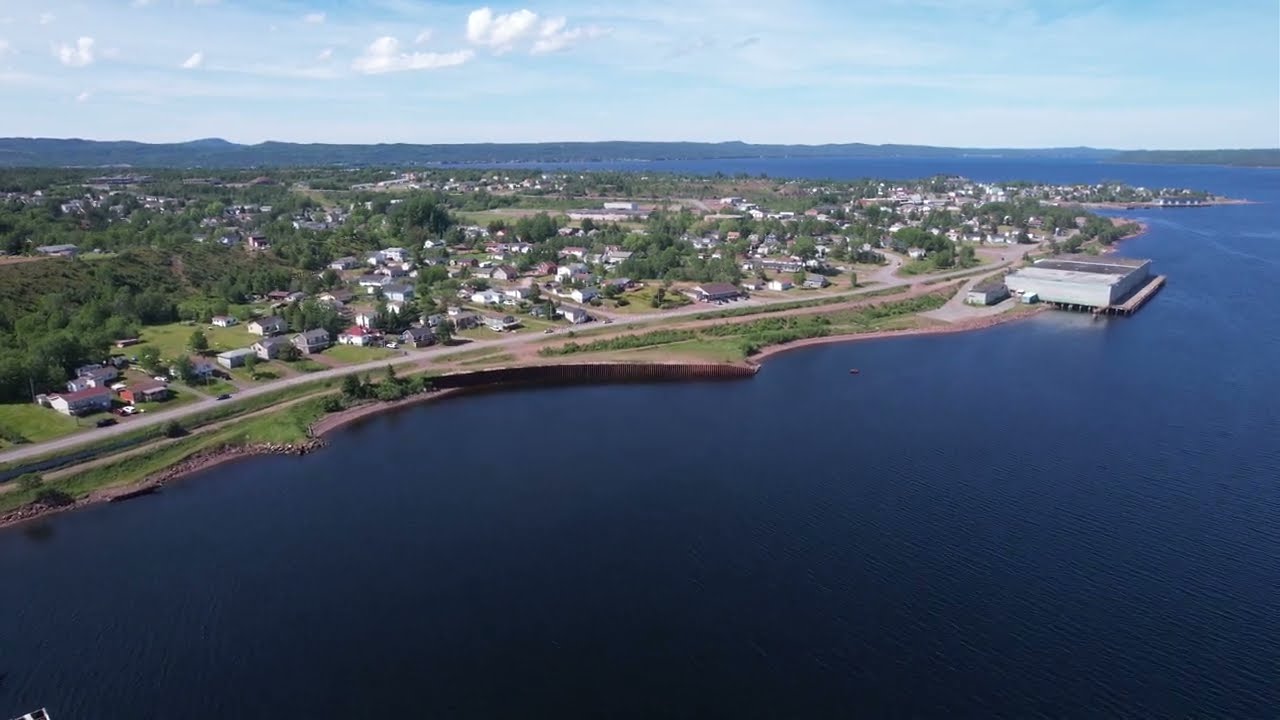This aerial image captures a picturesque small town nestled along the shoreline of a large, dark blue body of water, possibly a lake or river. The water appears empty and contrasts beautifully with the vibrant, light blue sky above, dotted with wispy white clouds spanning the horizon. The town's coastline, featuring an orangey-brown tint, transitions into lush green grass and shrubs interspersed with a few trees.

Dominating the right-hand side of the shoreline is a large, grey, and possibly white building with a black roof, extending slightly over the water with a platform. This building is accessible by a road running parallel to the water's edge. The town includes a mix of white houses, some with dark grey or red roofs, surrounded by greenery, creating a tapestry of suburban and natural elements.

A prominent road cuts through the town, along the water, leading to various suburban clusters and barrier protections around the town's water boundary. The backdrop features a range of hills or mountains, painted in dark bluish-brown tones, stretching across the entire width of the image, completing the idyllic scenery with additional wooded areas beyond the immediate town.